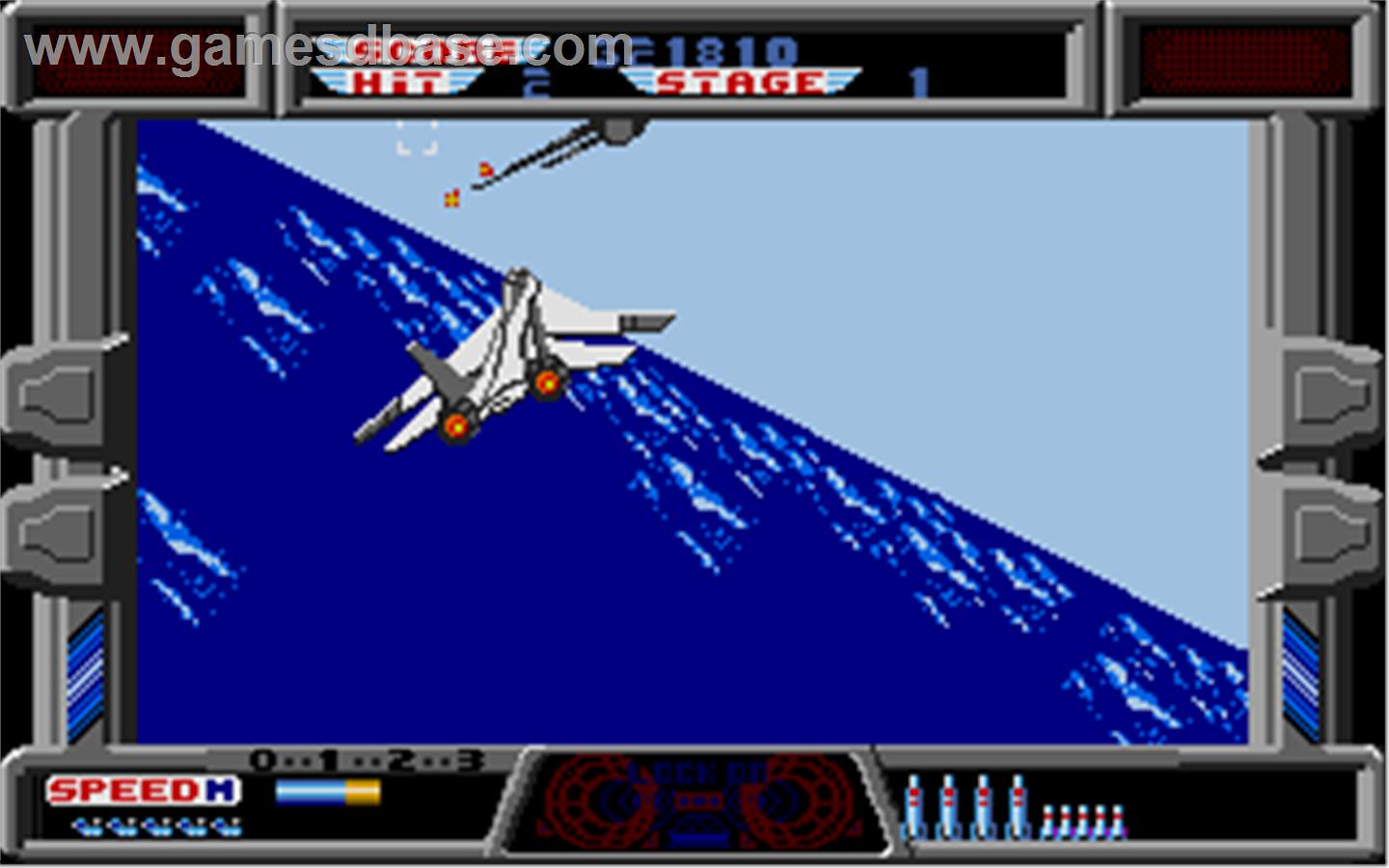This detailed depiction presents a scene from a video game featuring a military jet aircraft soaring over a body of water. The water is depicted with varying shades of blue, accented with light blue and white textures at the top to simulate the patterns of waves. The airplane, resembling an arrowhead, is characterized by its sleek, aggressive design with swept-back wings and dual tail fins. It is equipped with two jet engines, each mounted under a tail fin, and the cockpit appears to be narrowly constructed, presumably holding one or at most two occupants, reflecting its military use.

The sky above the water is a medium blue, further immersing the viewer into the flight simulation environment. Additionally, another unidentified object with black and orange hues is visible in the sky, adding an element of intrigue.

The image is framed by a black border. In the top left corner, the website "www.gamesdbase.com" is clearly legible. There are various in-game indicators and information presented in red, white, blue, and yellow colors, providing essential details to the player.